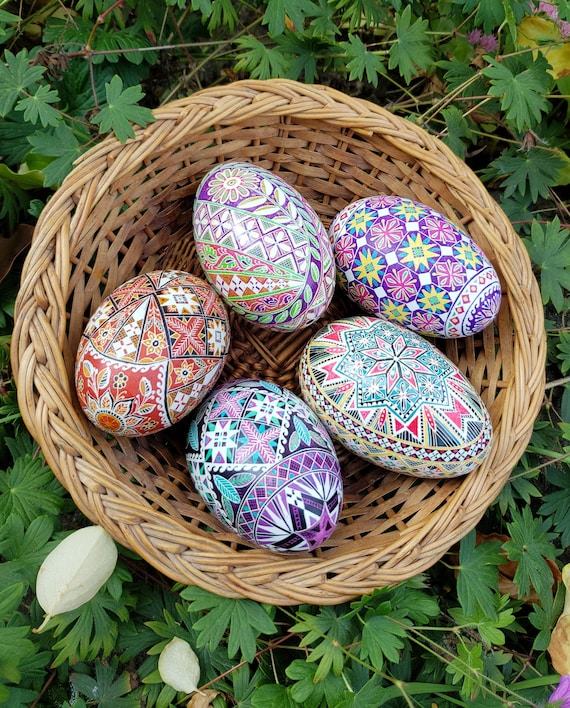The image features a close-up, aerial view of a wicker basket containing five beautifully hand-painted eggs, set against a lush, green backdrop of leafy vegetation reminiscent of ground cover. Each egg, larger than the average size, showcases a multitude of vibrant colors including purple, pink, green, yellow, red, blue, orange, and gray. The eggs have intricate, varying designs with patterns such as spirals, diamonds, and crosses, with each egg predominantly displaying a unique color scheme—one leaning more towards red, another towards pink, while others have greenish or bluish backdrops, and one is a blend of all hues. The scene is reminiscent of a delightful Easter arrangement, enhanced by the contrasting greenery that frames the basket, creating a picturesque and enchanting setting.